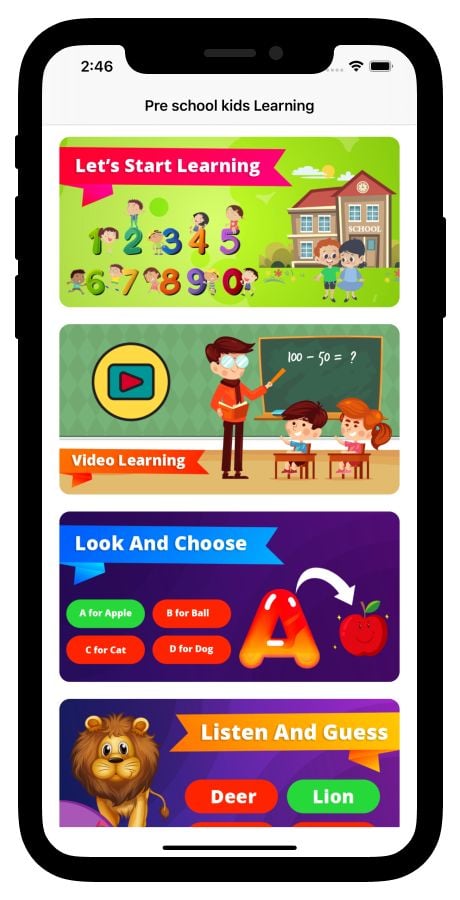This image captures a phone interface displaying several educational options at 2:46 (unspecified whether a.m. or p.m.). The phone shows full Wi-Fi connectivity and a fully charged battery. The top section, titled "Let's Start Learning," features vibrant graphics with numbers 1 through 10 and animated children climbing over them. In front of the numbers, there are male and female teachers, and a school building is visible in the background.

Below this, there is an option named "Video Learning." It is illustrated with a play symbol, a boy and a girl seated at their desks, and a teacher pointing to a whiteboard with a ruler. The whiteboard displays "100 - 50 =" followed by a question mark.

The next option is "Look and Choose," which visualizes letters A to D with corresponding pictures: A for Apple, B for Bell or Ball, C for Cat, and D for Dog. An arrow points from the letter A to an apple.

The last visible option is "Listen and Guess," showing an image of a lion with multiple-choice answers including deer and lion, although the third option is cut off. Both the "Look and Choose" and "Listen and Guess" sections are highlighted in green, indicating correct selections.